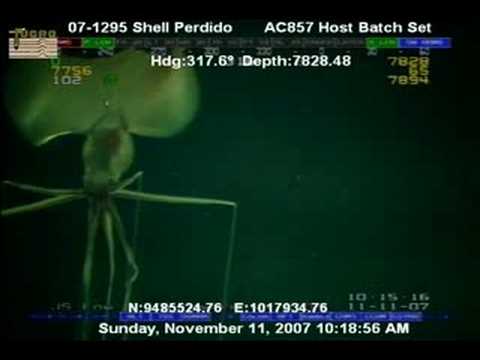The image, captured in a small horizontal rectangle, displays detailed informational overlays on a dark greenish background. Dominating the left side is an image that resembles a green bug or aquatic creature, its body marked by two larger translucent, almost jellyfish-like rounded sections on the top and a smaller rounded section below with a dark spot and a protrusion. From the central body, six to eight long legs project in various directions: three or four in the middle, two extending leftward, and one sharply bending to the right.

White text across the top reads: "07-1295 Shell Perdido AC857 Host Batch Set." Below this, additional details include the text "HDG: 317.6° Depth: 7828.48." Some faint numbers and letters are visible behind this main text. On the right side of the image, green and blue bars with orange numbers are faintly visible. At the bottom center, the overlay displays the date "Sunday, November 11, 2007," followed by the precise time "10:18:56 AM," along with additional faint writings and numbers that seem to exist beneath the main white text. These details suggest the image might have been taken with specialized equipment, possibly under low light or night vision conditions.